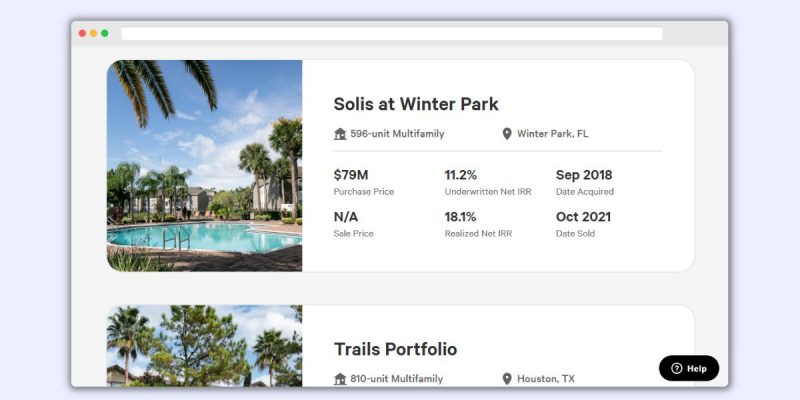This image features a detailed mock-up of a website for "Solace at Winter Park," a multifamily residential property. Prominently displayed is information indicating that this property consists of 598 units. An adjacent house icon reinforces its residential nature. On the left side, the location "Winter Park, Florida" is specified.

At the top of the image, several key data points are presented. The purchase price of the property is highlighted as $79 million. An important financial metric, the underwritten Internal Rate of Return (IRR), is prominently noted as 11.2%.

Further down, the image details the timeline of the investment. The property was acquired in September 2018. The acquisition price is listed as $18.1 million. The realized Internal Rate of Return (IRR) is marked as being achieved in October 2021, which is also indicated as the date the property was sold.

Additionally, at the bottom of the image, there is mention of the "trails portfolio," and a picture of another property related to this portfolio is visible.